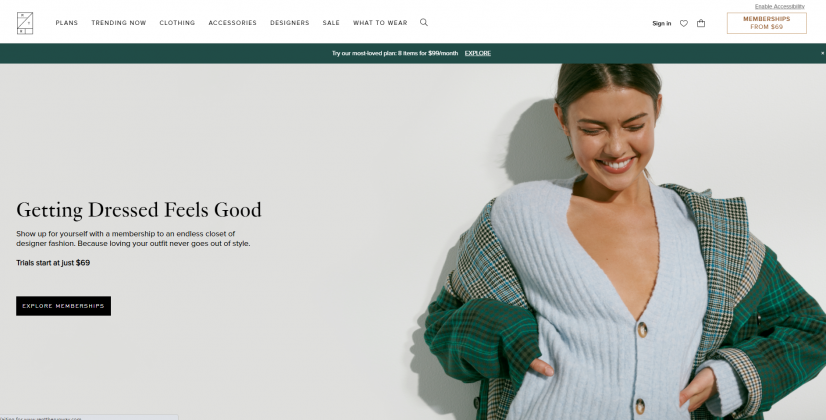The screenshot captured is of the homepage of a clothing website, boasting a sleek design with a light gray background. Dominating the right side of the screen is a vibrant image of a youthful model, who exudes charm with her warm smile and crinkled, closed eyes. The model, sporting medium-length brown or black hair tied back, is the epitome of fashion in a low-cut powdered blue button-up shirt. This shirt, adorned with two light tan buttons streaked with dark brown, speaks of subtle elegance.

Draped casually over her shoulders is a green plaid jacket, hinting at a layering trend with lighter colors underneath, maintaining the plaid pattern. The image leaves no doubt that these stylish pieces are available on the website.

On the left side of the screen, the website's tagline, "Getting dressed feels good," stands out in bold black text. Beneath it lies a brief description of the site's offerings, accompanied by a rectangular button with a black background, inviting interaction.

At the top, a white background menu bar with clearly readable black text ensures easy navigation. The upper left corner proudly displays the website's icon, a distinctive rectangular shape with a diagonal line cutting through it, symbolizing the brand's unique identity.